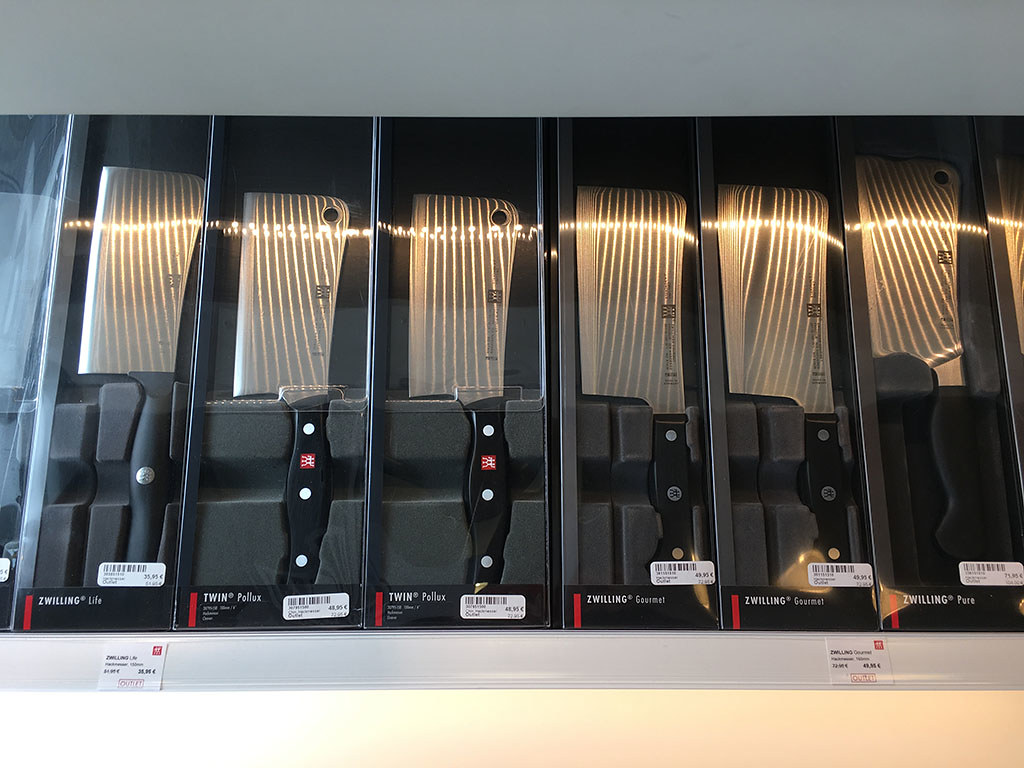This image showcases a collection of six Zwilling-brand cleaver-style chef knives, neatly displayed in plastic casing with clear tops. The first knife, labeled "Zwilling Life" and priced at $35.95, features a basic black handle with a single silver dot. Next are two "Twin Pollocks" knives, each priced at $48.95, with sturdier black handles adorned with three silver dots and a little red logo. These knives also have a distinctive hole in the top-left corner of their blades. Following these are two "Zwilling Gourmet" knives, similarly priced at $48.95, with broader blades and black handles featuring three silver dots and a gray emblem. The final knife, named "Zwilling Pure" and priced at $75.95, has a shorter but seemingly sturdier black handle with three dots. All knives have sharp silver blades and are packaged in boxes with the Zwilling logo—black with white lettering and a red bar to the right. The layout displays the knives from right to left, emphasizing their subtle differences in handle design and blade features.